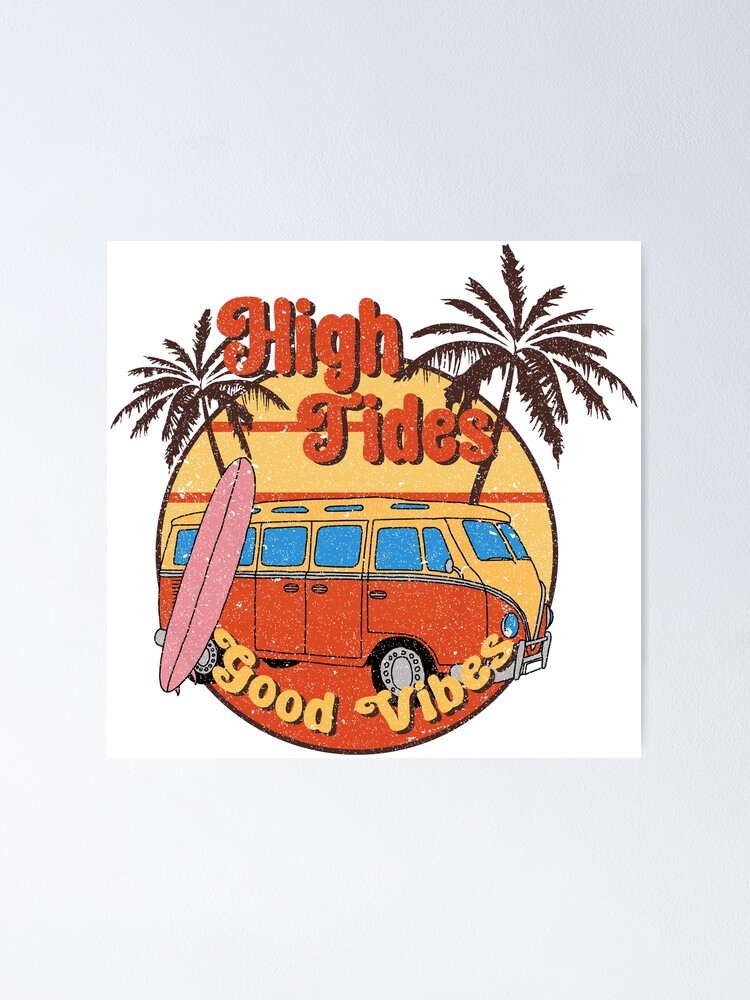This image is of a vintage-style sticker featuring an RV reminiscent of the classic VW bus. The sticker is set against a white square background, which appears to be stuck to a grayish-white wall. The central focus of the sticker is a round inset showcasing a vibrant scene.

At the top of the circle, in bold red font, it reads "High Tides," while at the bottom, in a yellow font, it says "Good Vibes." The RV is prominently displayed within the circle, painted yellow on the top and red at the bottom, separated by a blue stripe. The RV has blue windows, blue headlights, and silver hubcaps on black tires. A light pink surfboard, angled and leaning against the side of the RV, adds a touch of whimsical charm.

Flanking the RV are two palm trees protruding from behind, their brown trunks stretching up above the vehicle. The background within the circle is adorned with warm hues of yellow, orange, and light yellow stripes, giving it a classic 70s-80s groovy aesthetic. The overall distressed look of the sticker, combined with its vivid color palette, evokes a nostalgic and laid-back beach vibe.